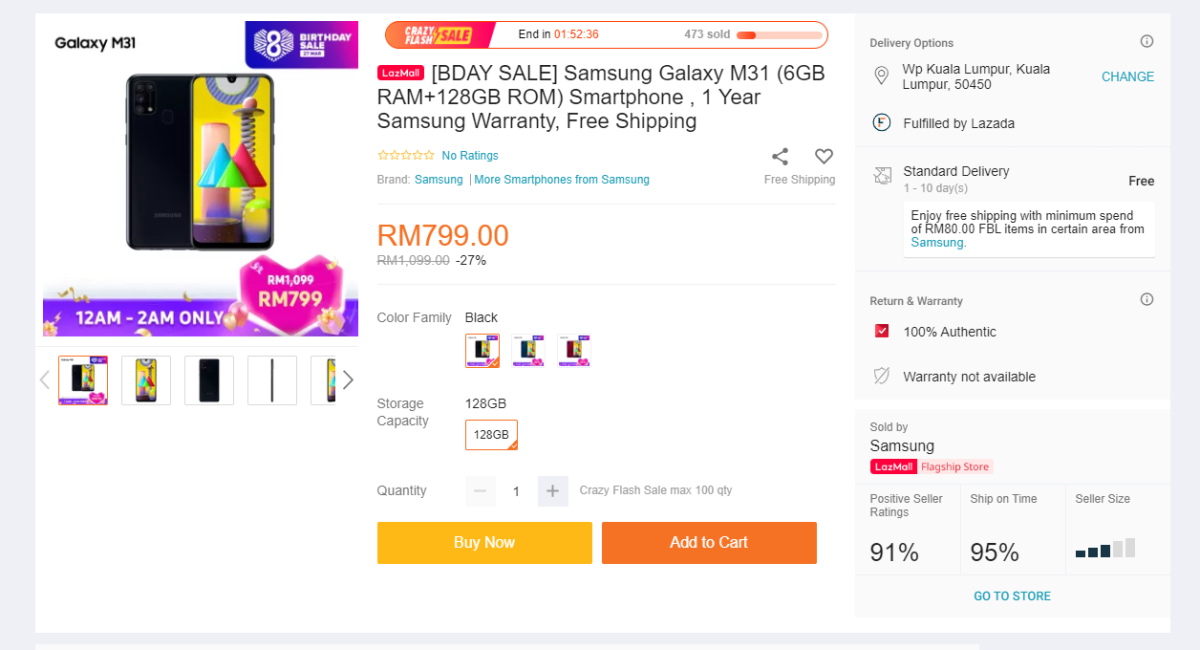The image depicts a website layout similar to e-commerce platforms like AliExpress. The background is gray on all edges (left, right, top, and bottom), while the central area is white. At the top left, black text reads "Galaxy M31". 

Centered at the top is a sale notification bar stating "Ends in 1 hour and 52 minutes and 36 seconds," accompanied by a progress bar indicating "473 sold" to the right. Below this, the product description "Bidet Sale: Samsung Galaxy M31, 6GB RAM, 128GB ROM, Smartphone, One Year Samsung Warranty, Free Shipping" is displayed. The price of the phone is listed as $7.99.

Below the price, there are "Buy Now" and "Add to Cart" buttons. On the right side of this section, delivery options, addresses, and delivery types are shown. Additionally, there are product ratings and a note that the item is sold by the "Samsung Flagship Store" in the bottom right corner.